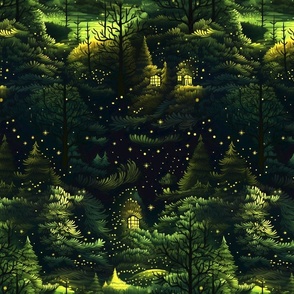This digital illustration is a square-shaped, magical nighttime scene set in a lush, dark green forest. The atmosphere exudes both an enchanting and slightly eerie vibe. The sky is barely visible, suggesting it is night, and the scenery is illuminated by scattered golden speckles resembling fireflies or magical dust floating through the air. 

Amongst the dense foliage, patches of bright yellow provide a striking contrast, resembling moonlight filtering through the thick canopy. The forest is peppered with numerous black silhouettes of tree trunks and branches, some of them bare and skeletal, adding to the mystical yet spooky ambiance. Additionally, there are several small houses with glass windows nestled within the forest, indicating perhaps a hidden community, possibly of elves. Three or four lanterns are also scattered around, providing subtle illumination that enhances the forest's whimsical charm.